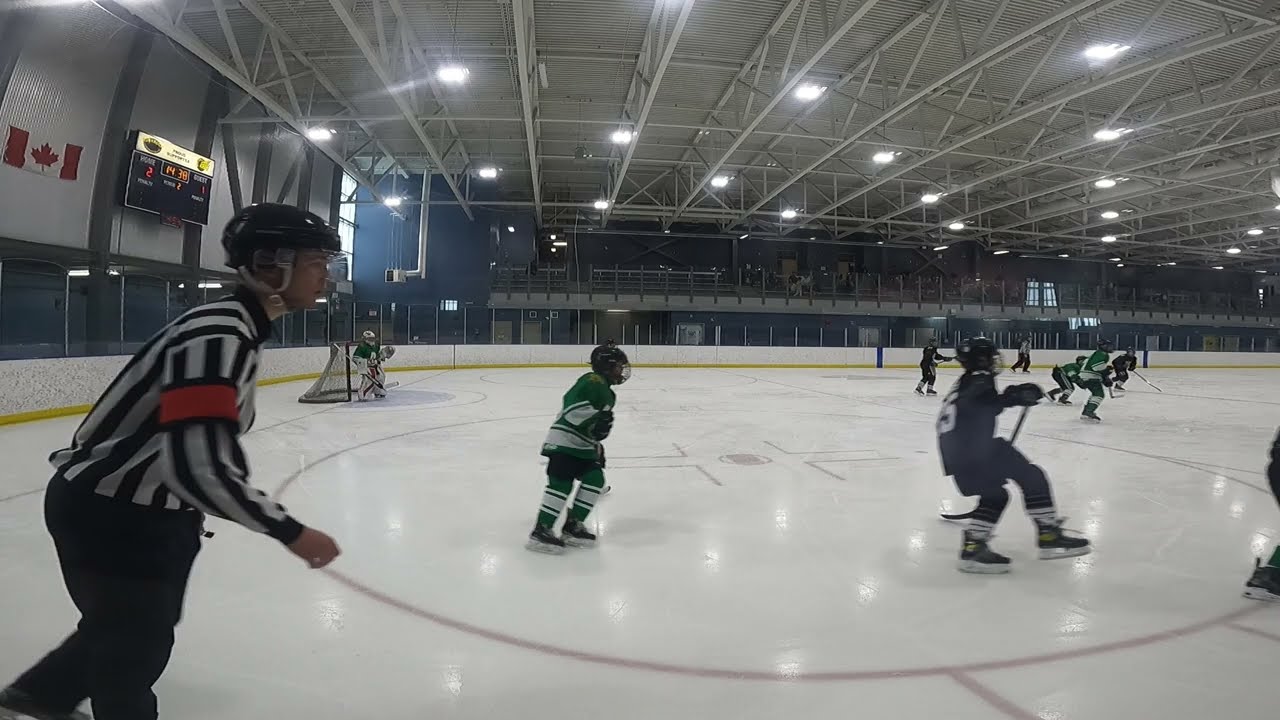In this image, a youth ice hockey game is taking place inside a large arena with a white roof and plexiglass panels surrounding the rink. The players, appearing to be young boys, are divided into teams wearing green and white jerseys and navy blue jerseys. At the forefront, two players are seen skating to the left with their sticks, and a referee dressed in a black and white striped jersey, black pants, a red armband, and a helmet is also visible. The scoreboard above indicates a score of 2-1, possibly in the second period with around 14 minutes remaining. Additional players are scattered in various stages of play, and a goaltender can be seen guarding the goal to the left. At the far end, a Canadian flag hangs on the wall, adding to the quintessential rink environment.